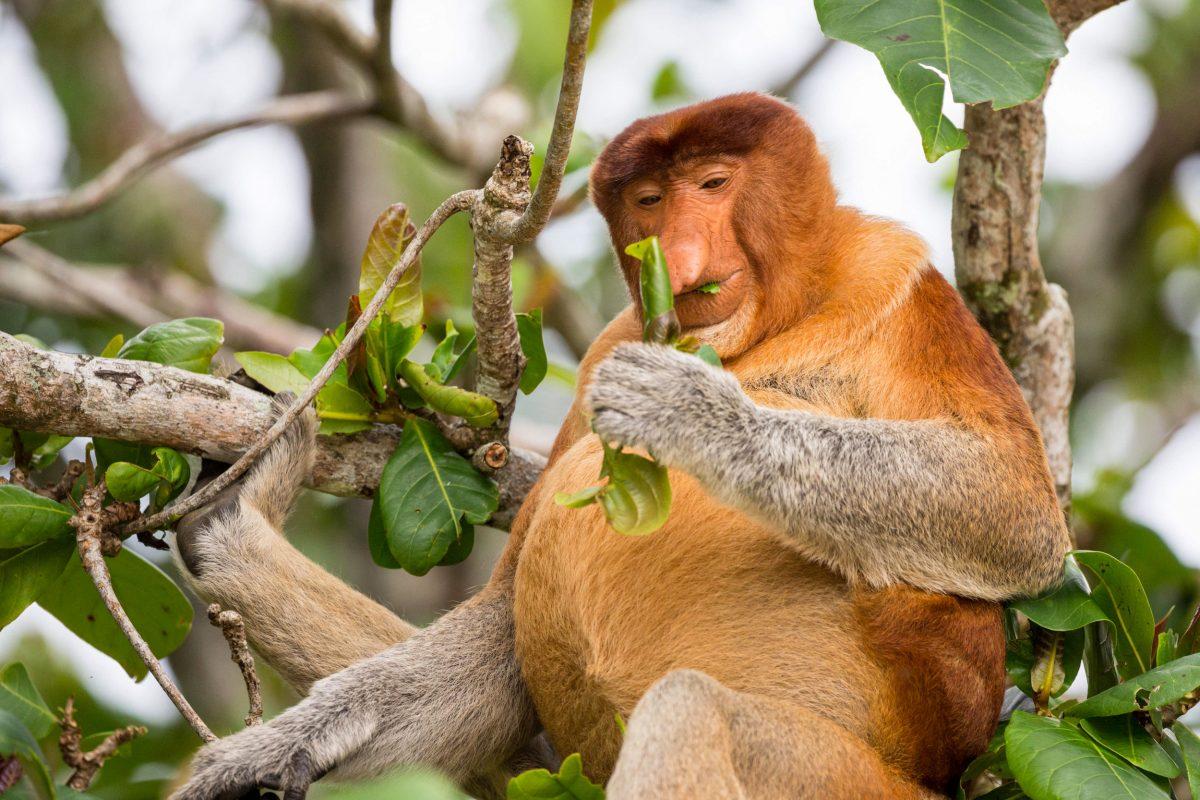In the blurred jungle background, dappled with sunlight and framed by an array of branches and leaves, sits a peculiar-looking baboon with a notably large, forked nose. Its face, which is relatively smooth with minimal hair, is surrounded by brown fur that transitions into darker shades on the shoulders. The fur on its arms and legs below the knees turns a grayish color. The baboon's potbelly stands out, light brown in hue, adding to its distinct appearance. Seated comfortably on the tree's branches, the baboon is holding a handful of green leaves, with one piece delicately hanging from its mouth. An intriguing object, possibly another limb, appears to grasp a nearby branch, adding an element of mystery to the scene.